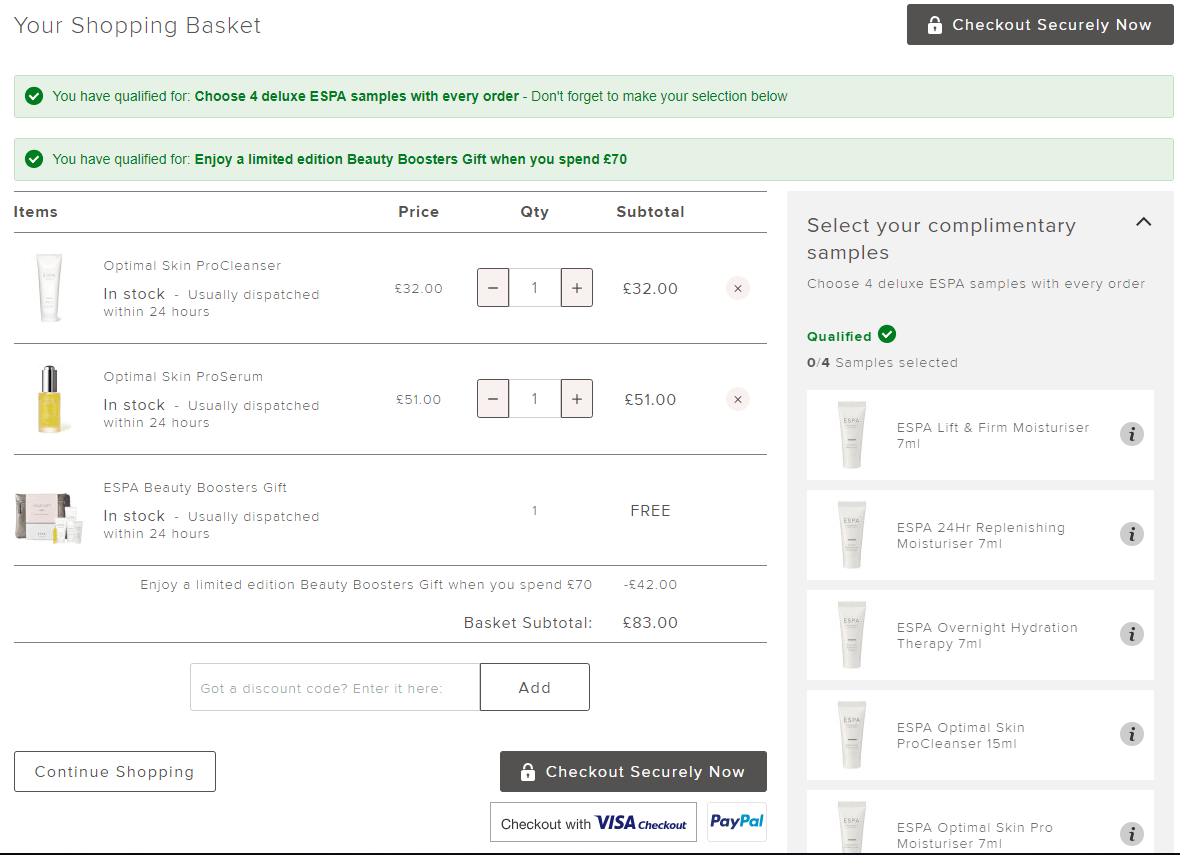This is a detailed overview of a shopping webpage for a cosmetic and facial products store:

The webpage features a prominent shopping basket icon located in the top left-hand corner, rendered in a subtly-colored font. Directly beneath this icon are two highlighted messages aimed at the shopper, each accompanied by a green checkmark. These messages serve as reminders or prompts, urging the shopper to pay attention to specific info, primarily functioning as advertisements or attempts to upsell additional products.

Adjacent to these messages, there is a black rectangular button emblazoned with a white lock icon and white text that reads "Check out securely now." This button acts as a hyperlink, directing users to the secure checkout page.

Below the highlighted sales prompts, the webpage follows a conventional layout typical for e-commerce sites. Displayed here are products that the shopper has already selected, complete with a running total of their cost. The site also showcases a range of suggested products, aiming to entice additional purchases. Overall, the page includes clear navigation tools for the customer to review their selections and proceed to payment.